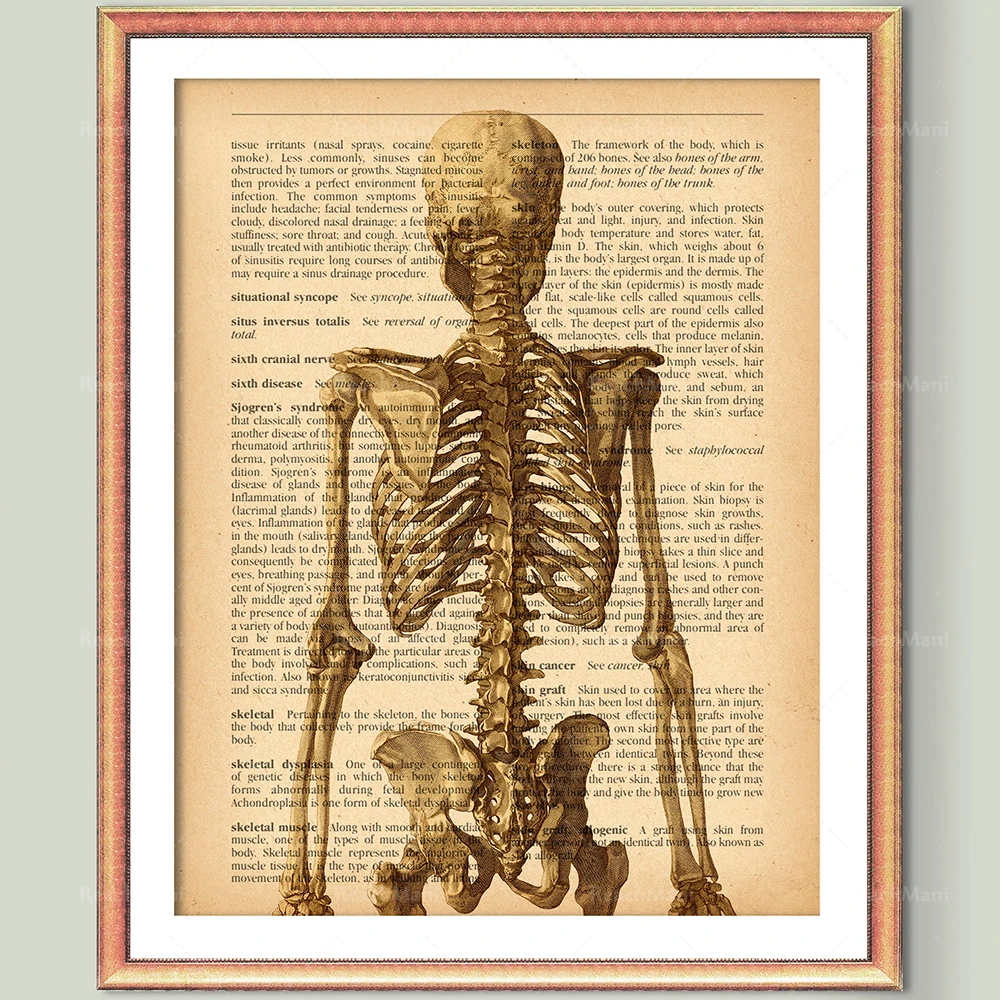The image showcases a detailed and intricate scene centered around a photo frame attached to a light gray, olive-tinged wall. The frame itself is a complex blend of reddish-brown hues and faded beige, adding a rustic charm to the composition. Inside the frame, a narrow white border elegantly outlines a piece of paper resembling an old, tan pirate map. This paper, light brown in color, prominently features a translucent brown human skeleton viewed from the back, revealing the back of its head and spine. Surrounding and overlaying the skeleton are numerous paragraphs of small black text, which seem to be of a medical nature. Highlighted words such as "situational syncope," "situs inversus totalis," "sixth cranial nerve," "sixth disease," "Sjogren's syndrome," "skeletal dysplasia," "skeletal muscle," "skeleton," "skin," "skin cancer," and "skin graft," indicate the text's comprehensive medical focus. The meticulous layout and the overlapping elements create a visually engaging and informative display.